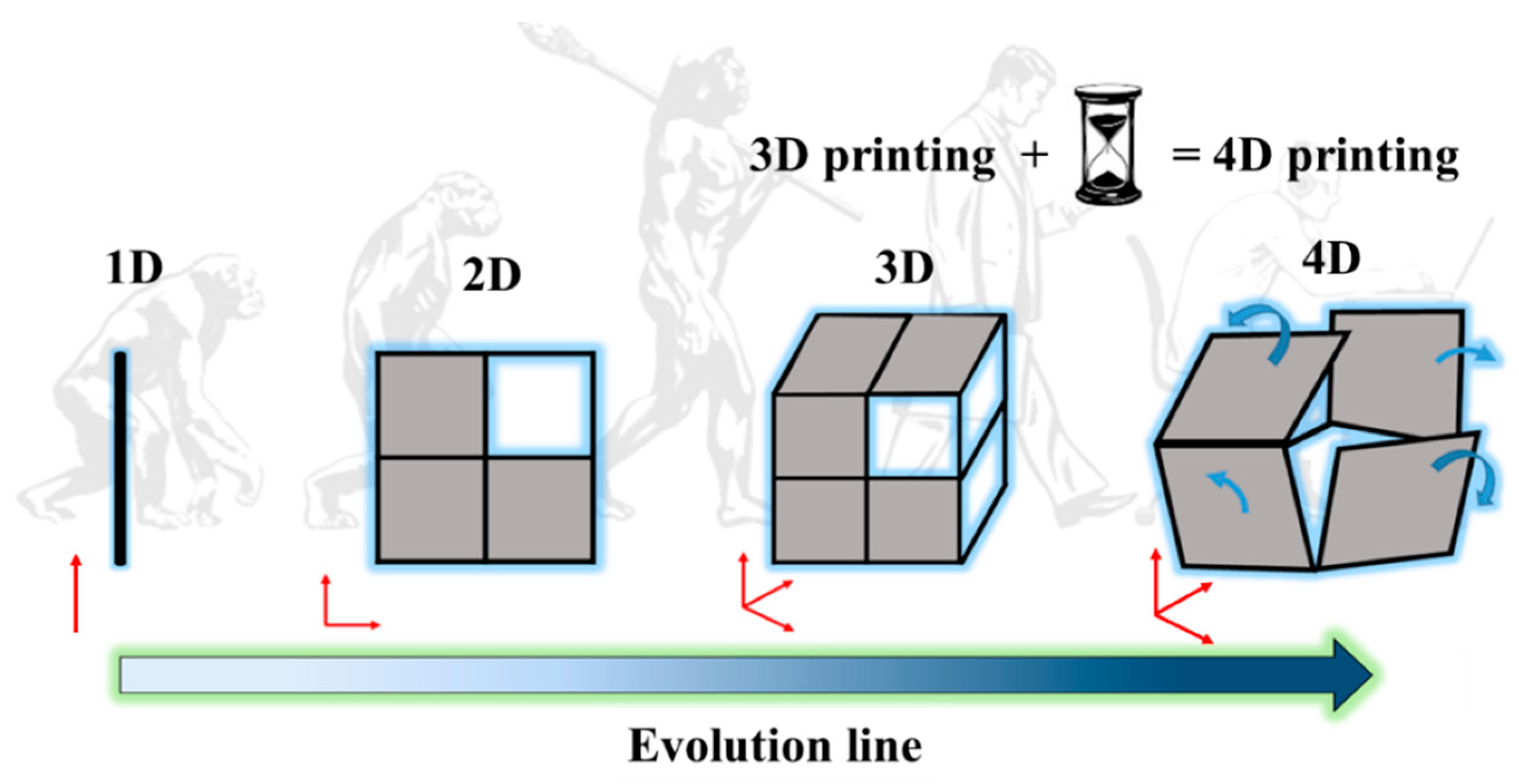The image is a detailed diagram illustrating the evolution of dimensions and the concept of 4D printing. The backdrop features a classic evolutionary sequence, starting with a monkey on all fours, followed by a progressively upright ape, a Neanderthal, a modern man in a suit, and finally, a man seated at a computer.

Superimposed over this evolutionary background is a sequence of images representing different dimensions. On the left, labeled "1D," is a single line over the monkey. Moving right, "2D" is depicted with a square over the upright ape. "3D," shown as a cube, is placed between the Neanderthal and the modern man. The "4D" image, over the seated man, features a box that appears to be unfolding, symbolizing the fourth dimension, often interpreted as time.

Text at the top of the diagram states, "3D printing + hourglass = 4D printing," linking the concept of 3D printing with the element of time to explain 4D printing. Below this text, arrows indicate progression: a simple upward line under "1D," an L-shaped line under "2D," a more complex three-dimensional line under "3D," and an even larger, similar line under "4D." At the bottom, a large arrow labeled "evolution line" runs horizontally from "1D" to "4D," emphasizing the progression through dimensions. The overall image combines these visual elements to communicate the advanced concept of 4D printing through the analogy of dimensional evolution.